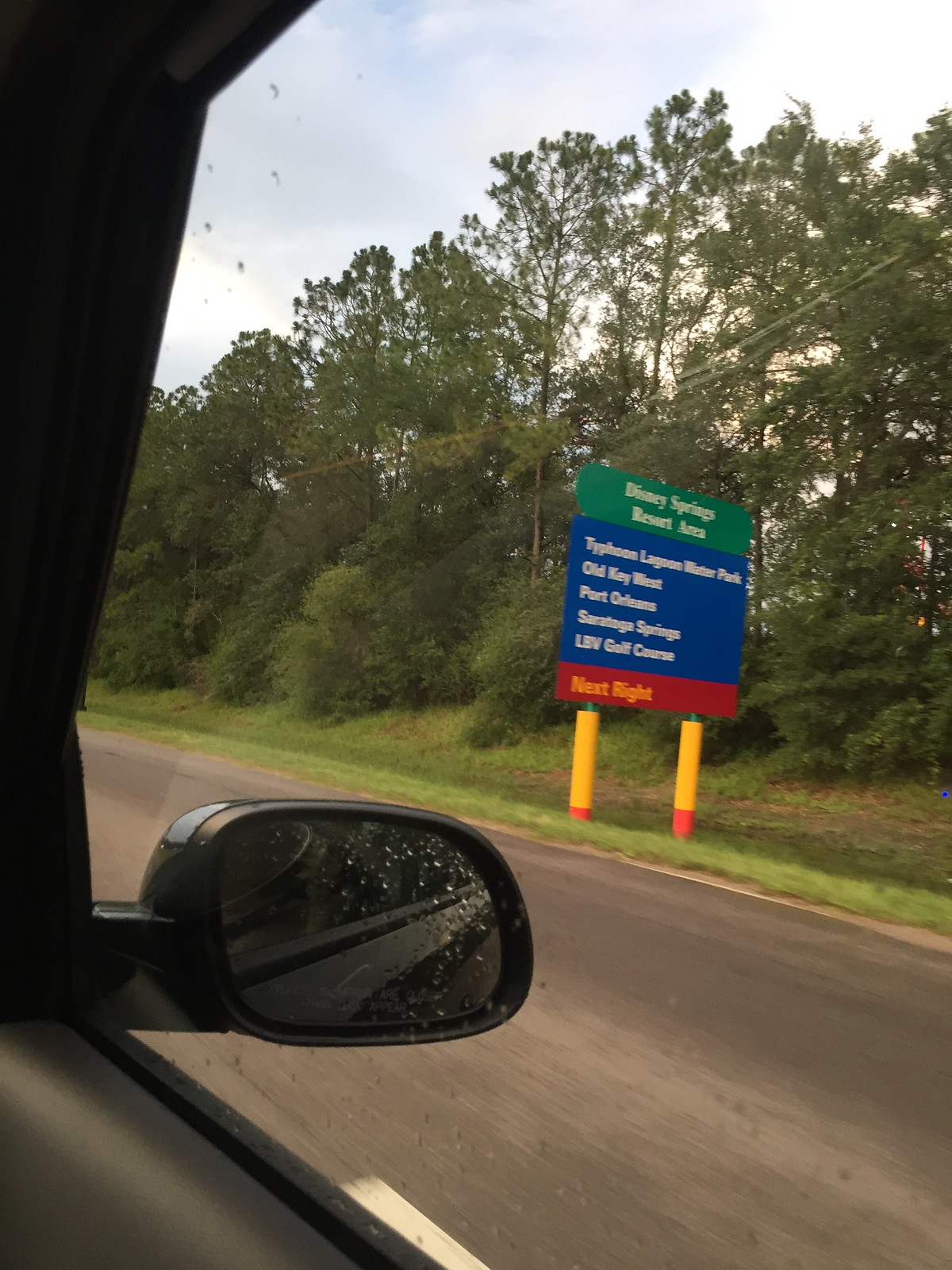This color photograph is taken from inside a vehicle, likely the passenger seat, capturing an external view through the window on a greyish road with a focus on a large, colorful sign. The sign, which stands out prominently against a backdrop of lush greenery and towering trees, is supported by two yellow poles with red bases designed to be highly visible. The sign, divided into three segments, features green, blue, and red backgrounds from top to bottom, each segment with white text. The top section reads "Disney Springs Resort," while the blue middle section lists several attractions, including "Typhoon Lagoon Water Park," "Old Key West," "Port Orleans," "Saratoga Springs," and "LBV Golf Course." The bottom red section indicates an upcoming turn with "Next Right." This detailed scene is further accentuated by raindrops visible on the vehicle's side window and rearview mirror, adding a touch of post-rain ambiance to the overall setting.